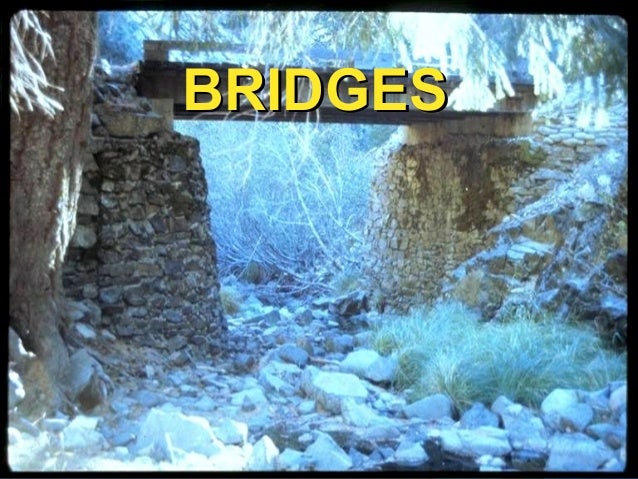This outdoor image is presented within a thin black border, reminiscent of a picture frame with rounded corners, adding a vintage or slide-like feel. Dominating the image is a stone bridge, constructed with large stone bricks and blocks, featuring a cement top with a traditional guardrail and steel girders. The bridge itself crosses over a rocky path, flanked on both sides by rocky cliffs adorned with moss and patches of grass. White tree branches, heavily laden with snow, cascade from the upper left corner, adding to the wintery atmosphere, with snow dusting the large rocks and boulders below. At the background, more snow-covered tree branches hang, creating a scene that is both serene and rugged. Central to the image, written in bold, bright yellow font, the word “BRIDGES” stands out, both an anchor to the composition and a title that gives context to the wintry, stone-laden landscape.